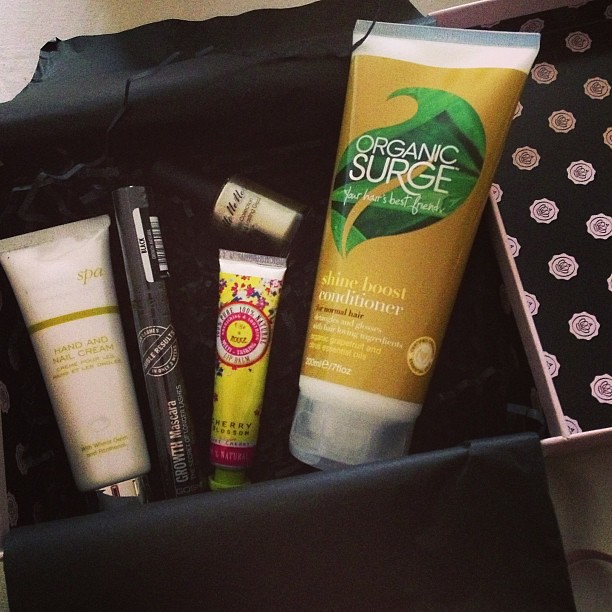This is a full-color photograph, likely taken indoors, featuring an open beauty subscription box with a sturdy, heavy-stock exterior. The inside of the lid is black, adorned with pink medallions bearing crown logos, repeated in a decorative pattern. Inside the box, black tissue paper is used as a liner. The contents include five different beauty products: 

1. A large yellow tube labeled "Organic Surge Shine Boost Conditioner" with a green leaf graphic.
2. A smaller yellow tube with purple printing, which says "Cherry Blossom."
3. A white squeeze bottle for hand and nail cream with a black lid.
4. A black tube of Growth Mascara with silver writing.
5. A glittery silver nail polish in a glass bottle with a black lid.

The arrangement of the items within the box emphasizes both the variety and the aesthetic appeal of the beauty products.